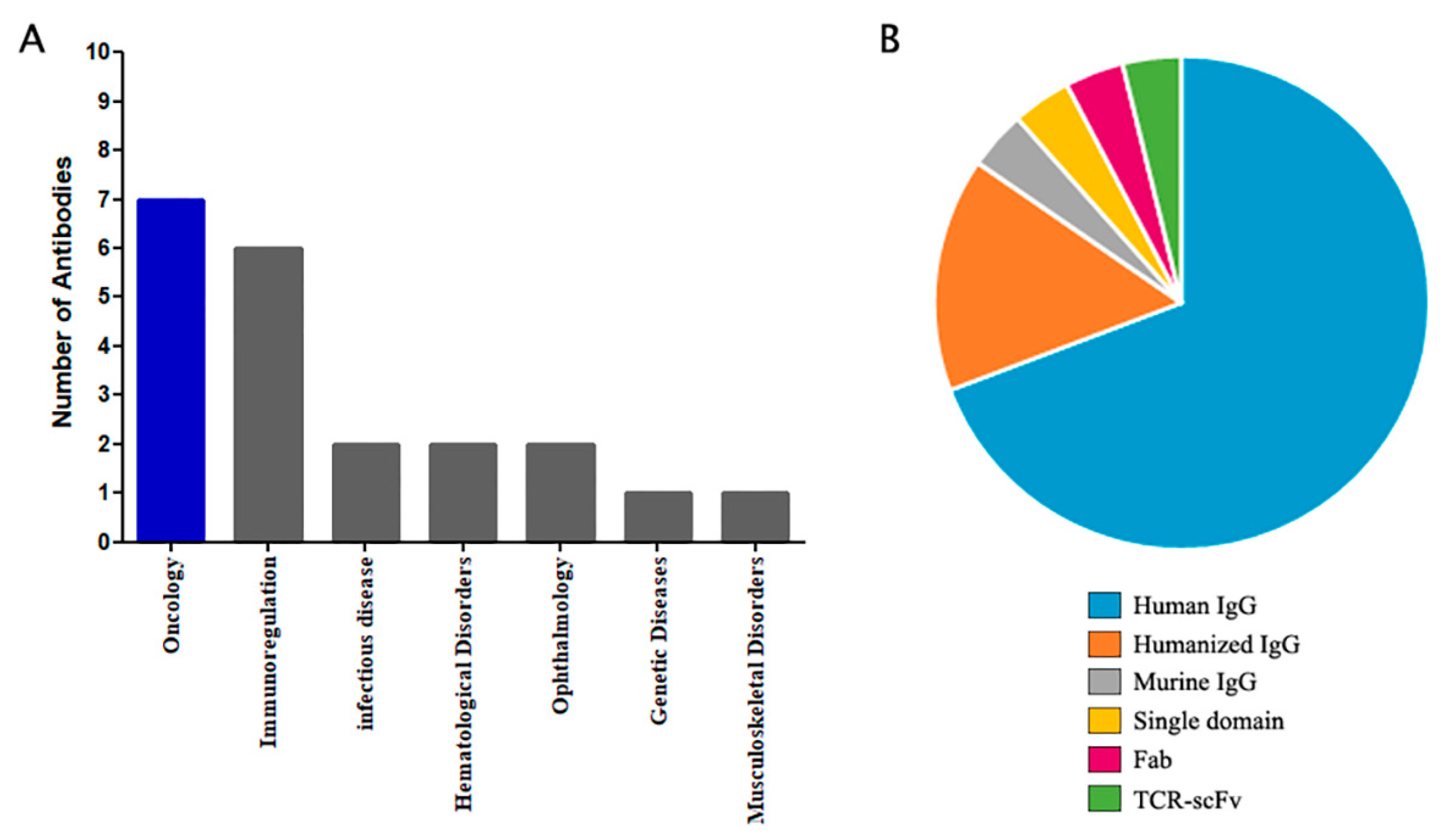The illustration presents two types of charts: a bar chart labeled 'A' on the left and a pie chart labeled 'B' on the right. The bar chart measures the "Number of Antibodies," with a vertical axis ranging from 0 to 10. It categorizes data across various medical fields displayed horizontally, including Oncology, Immunoregulation, Infectious Disease, Hematological Disorders, Ophthalmology, Genetic Diseases, and Musculoskeletal Disorders. Notably, Oncology leads with a blue bar reaching up to 7, while Immunoregulation follows with a height of 6. Infectious Disease, Hematological Disorders, and Ophthalmology each reach 2, and the remaining categories measure 1. 

The adjacent pie chart is dominantly blue, representative of Human IgG. It also includes significant orange (Humanized IgG) and smaller segments in gray (Marine IgG), yellow (Single Domain), pink (FAB), and green (TCR SCFV). Each color is defined in a key below the charts. The visual aid is digitally presented with vibrant pastel hues, enhancing the clarity and distinguishability of the data segments and categories.